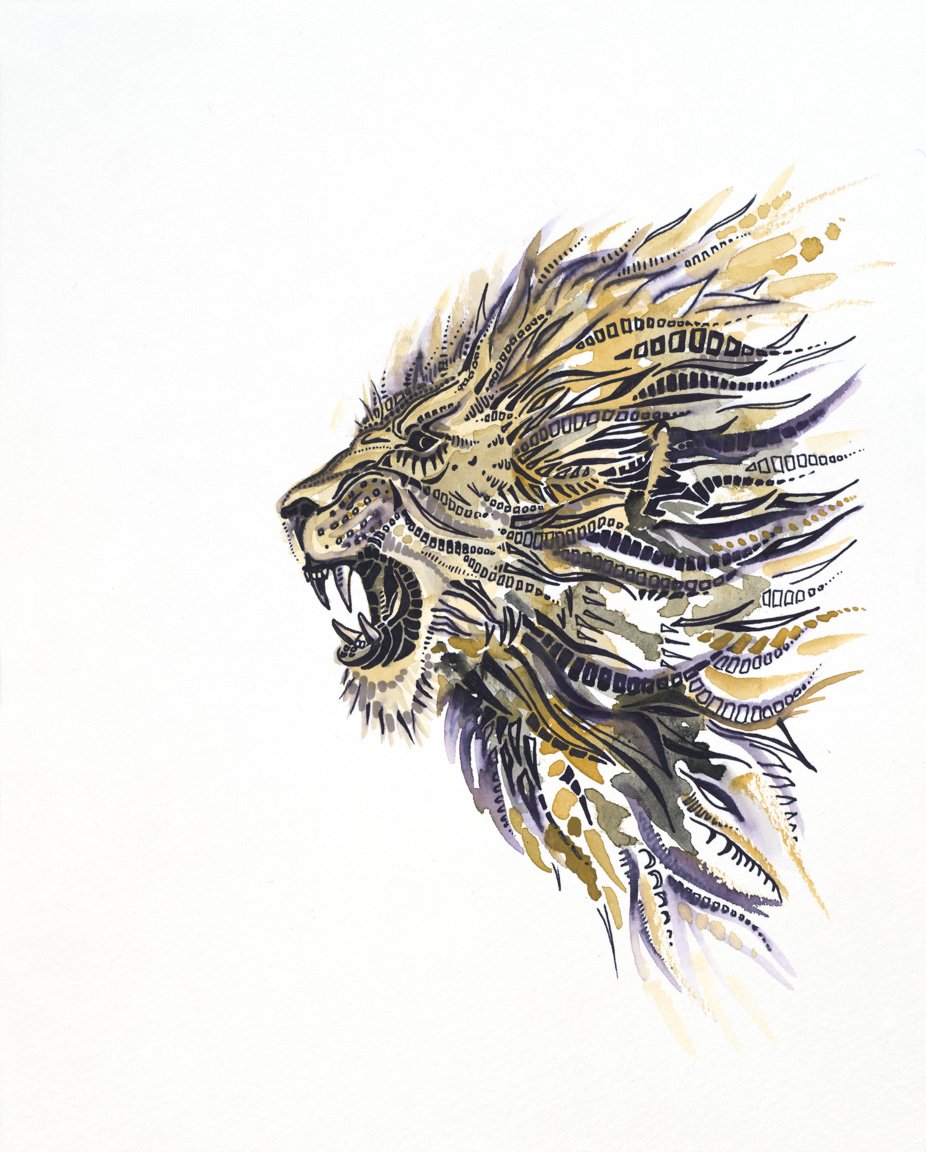The image is a detailed watercolor illustration of a male African lion's head, portrayed in a portrait orientation against an off-white gray background. The lion is facing left, showcasing one eye, part of its nose, and an open mouth revealing large incisors, giving it a fierce, prowling expression. The lion's face is predominantly a light beige or yellowish-tan color, accented with geometric designs and patterns in black pen. The mane, rendered in a combination of golden hues and deep purple accents, resembles feathers blowing in the wind. The intricate mane broadens towards the right-hand side of the image, adding dynamic movement and depth. Overall, the artwork combines bold color washes with meticulous pen detailing to create a striking, textured depiction of the majestic predator.